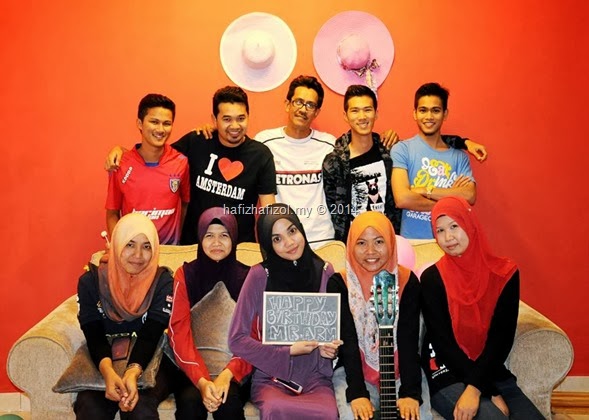This image features a vibrant group photo set against a bright orange wall, with a total of ten individuals. In the back row, five men stand closely together, their arms mostly wrapped around each other's shoulders, except for the man on the far right who has his arms crossed in front of his chest. One man is notably wearing a black shirt that reads "I Love Amsterdam." Above them on the wall, there are two women's hats mounted, one white and the other lavender.

Seated in front on a tan couch are five women, all wearing headscarves or veils. The woman in the middle holds a small chalkboard sign that says "Happy Birthday Mr. Arm," suggesting a celebratory occasion. To her left, one woman holds a pillow, and to her right, another woman holds an acoustic guitar. The rightmost woman on the couch has her arms folded in her lap. The image also faintly displays the text "HafizHafizal.my" in the center, with a copyright note dated 2014, indicating the likely source and date of the photo. The diverse group, possibly of Indian or Middle Eastern descent, is collectively wishing Mr. Arm a happy birthday in this colorful and warm snapshot.